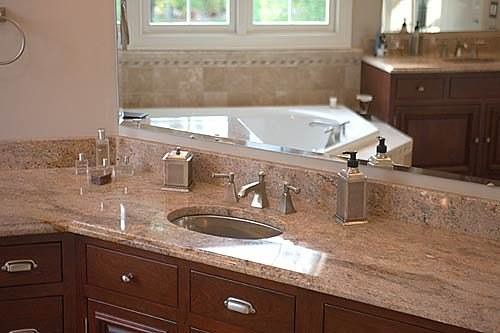This image showcases a well-designed, modern bathroom corner. The focus is on a sleek sink countertop that extends seamlessly into the corner, crafted with a dark wood base. The cabinetry below features an array of small drawers adorned with a mix of elongated silver handles and circular knobs, adding a touch of elegance.

The countertop itself is a rich blend of various brown tones, creating a sophisticated and earthy aesthetic. Nestled into this countertop is a circular sink, seamlessly integrated and complemented by a triangular faucet with dual handles for hot and cold water. Adjacent to the sink, a rectangular silver dispenser for lotion or soap and a matching silver box provide functional yet stylish accents.

In the large mirror mounted above the sink, the reflection reveals more details of the bathroom: a luxurious jacuzzi bathtub with clean lines, a portion of the countertop we are observing, and a crisp white double window that illuminates the space with natural light. Completing the countertop arrangement are several elegant glass bottles, enhancing the overall aesthetic of this meticulously designed bathroom corner.